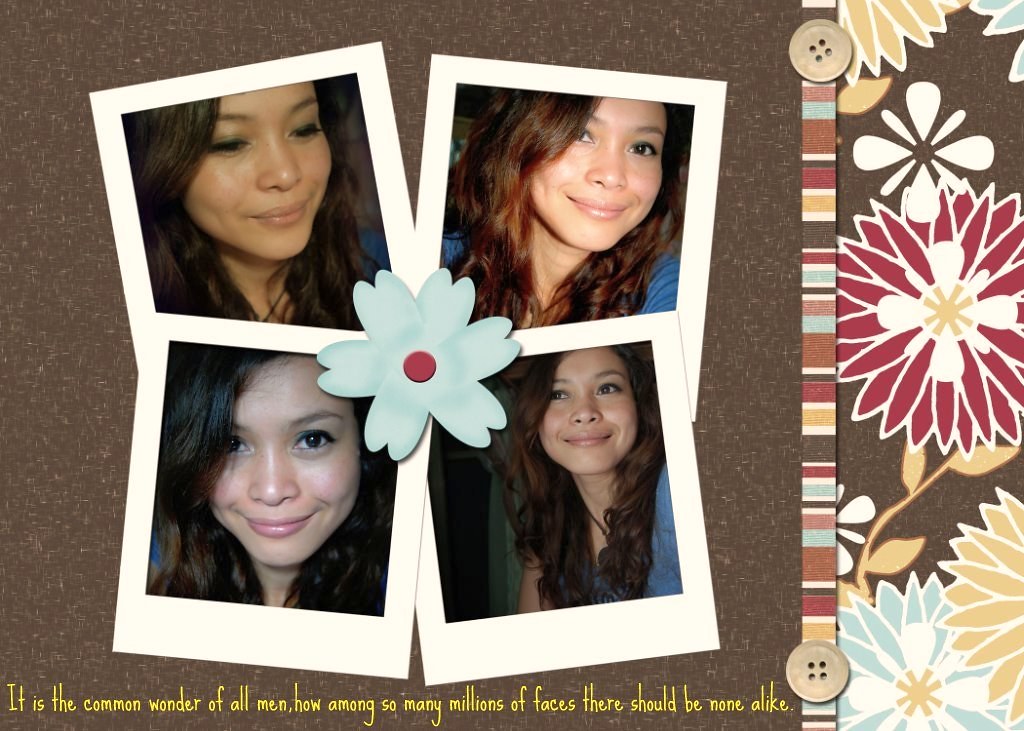The image depicts a cork board trimmed with multicolored fabric in hues of orange, blue, and maroon. Two taupe buttons are placed along the trim, accompanied by floral illustrations in muted tones of red, yellow, and blue. Central to the image are four Polaroid-style photographs of a woman with long, brown hair, wearing a blue long-sleeved shirt and smiling in different poses. These photos are arranged in a slanted square format and are pinned together by a white flower with a red center. Below the photos, in small yellow writing, the quote reads: "It is the common wonder of all men, how among so many millions of faces there should be none alike." The detailed background integrates elements of a cozy, cottagecore aesthetic, with a brown base that enhances the warm, inviting feel of the composition.